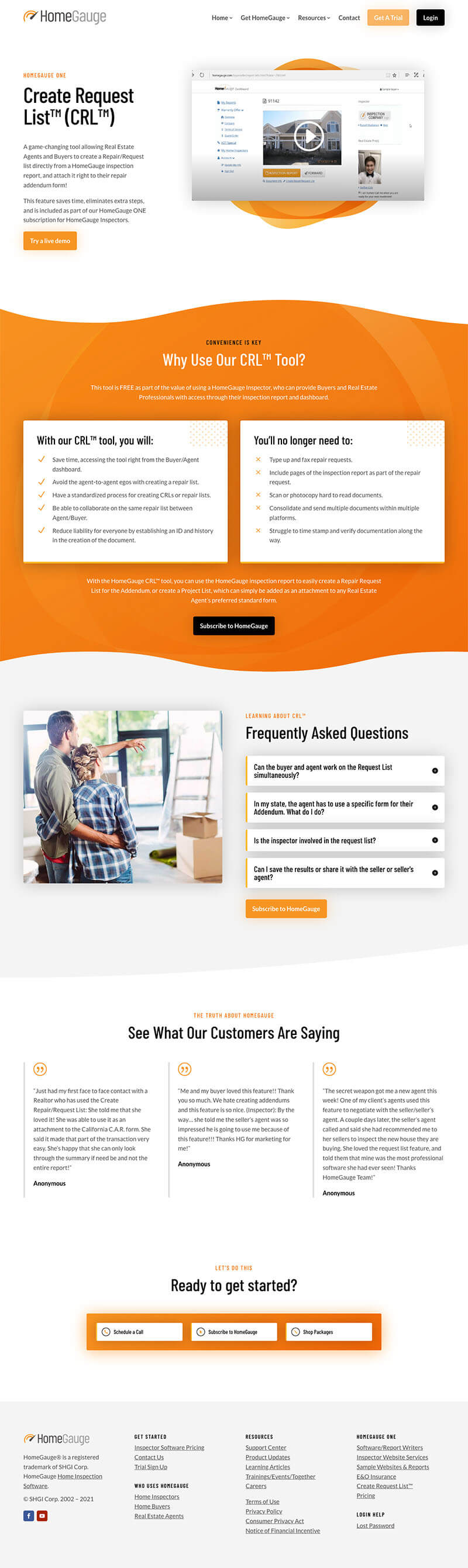**HomeGage Website Overview**

The HomeGage website serves as a comprehensive landing page featuring a variety of sections designed to inform and engage users about the company's services and tools. 

**Header Navigation**
At the top of the page, users can quickly access essential options such as "Home," "Get HomeGage," "Resources," "Contact," "Get a Trial," and "Log In." These navigation links ensure easy access to key parts of the site.

**Feature Highlight: Create Request List™ (CRL™)**
A major section is dedicated to one of HomeGage’s primary tools, the Create Request List™ (CRL™). This segment includes detailed information about the tool, complemented by a link to a live demonstration. Central to this section is an orange geometric rectangle that outlines the benefits of the CRL™ tool, underscoring its convenience. 

Two distinct text boxes within this section provide further insight:
1. **With Our CRL™ Tool, You Will:**
   - Multiple bullet points listing the features and benefits users can enjoy.
2. **You'll No Longer Need To:**
   - Bullet points detailing the tasks and hassles that the CRL™ tool can eliminate.

Additionally, a paragraph expands on the tool’s advantages, followed by a prominent "Subscribe to HomeGage" button.

**Frequently Asked Questions (FAQs)**
The next section addresses common queries with dropdown options that users can click to reveal answers. This segment is illustrated with a picture of a man and a woman examining a construction project inside a home, where everything is still boxed and wrapped. Another "Subscribe to HomeGage" button is positioned here for user convenience.

**Customer Testimonials**
To build trust and showcase credibility, there's a dedicated section for customer testimonials. Users can read three pieces of anonymous feedback praising the product. 

**Call to Action**
Towards the bottom, a compelling call-to-action strip invites users to take the next steps with text like "Ready to Get Started? Let's Do This." Users are provided options to schedule a call, subscribe to HomeGage, or shop packages.

**Footer Navigation**
The footer includes standard navigational links to help users explore the site further. This area covers topics like how to get started, the uses of HomeGage, available resources, HomeGage One, login assistance, social media handles, and registration information.

By structuring the content in this manner, the website effectively guides users through the various offerings and resources available, making it easier for them to find what they need.